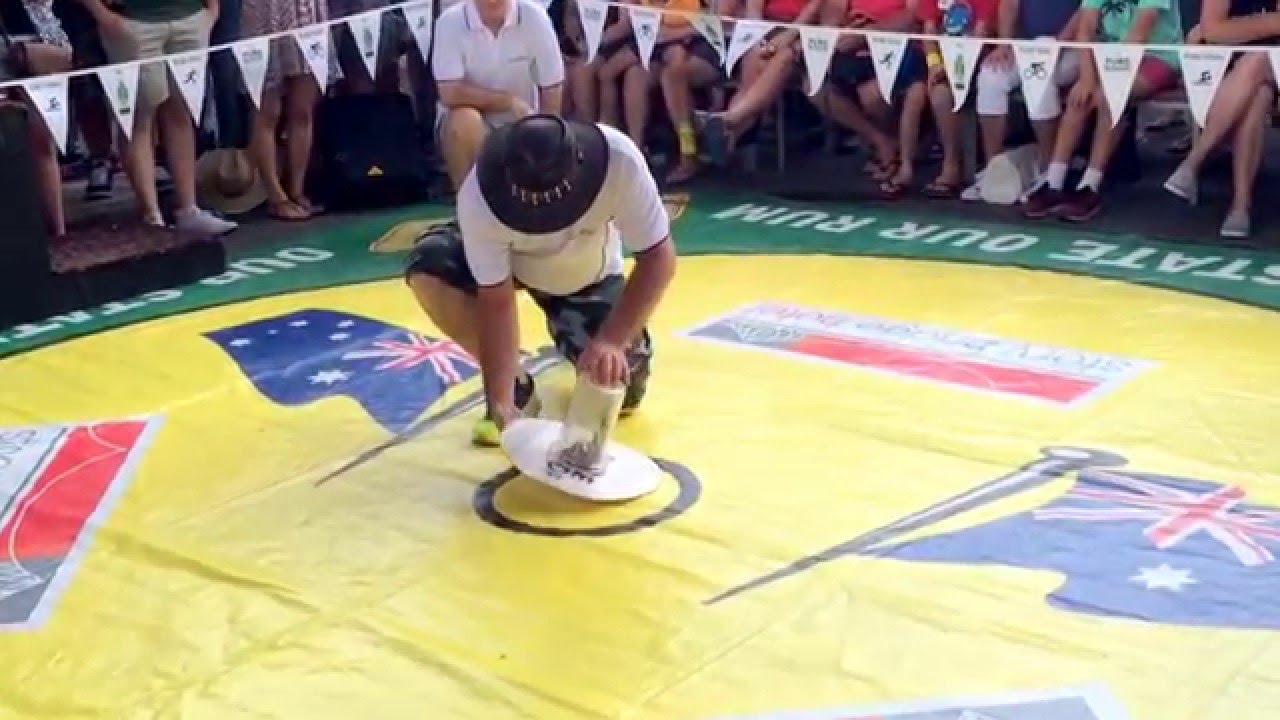This image depicts a man kneeling on a bright yellow mat adorned with various flag images, including Australian flags. He is positioned in the center of the mat, within a black circle. Wearing an Australian-style hat with detailing on the strap, a white t-shirt, and grey and black camouflage shorts, the man is carefully placing or lifting a conical glass canister within the black circle. There seems to be a small object inside the canister, possibly a snake, indicating some kind of capture-and-place competition. In the background, a crowd of spectators watches the event, while a man in a white polo shirt, likely a judge or referee, kneels behind the main participant. White pennant banners are also strung up around the area.